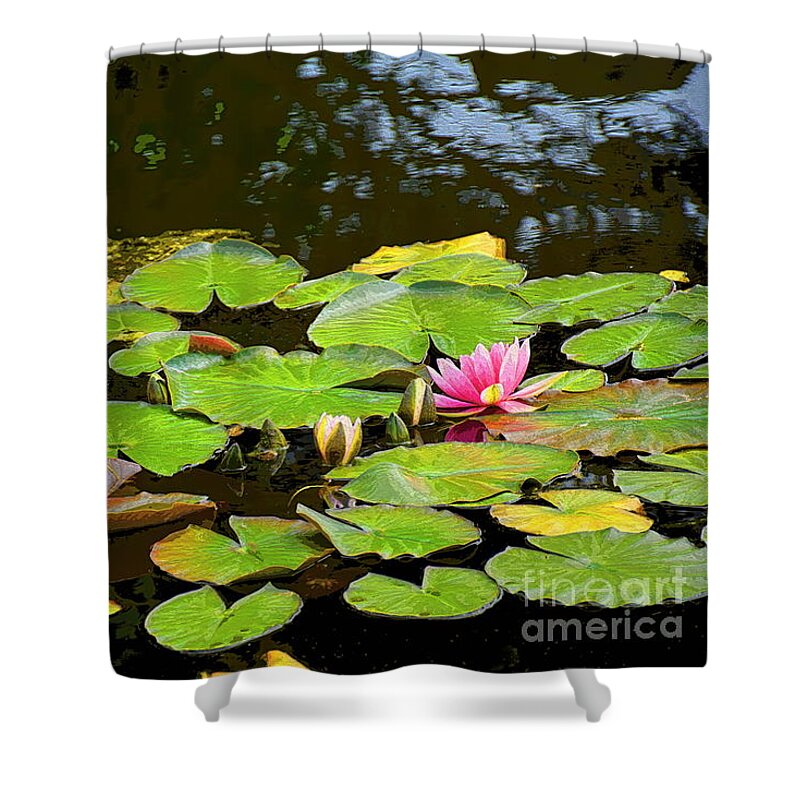The image shows a detailed depiction of a mock-up of a shower curtain with a design featuring a natural scene. The curtain has circular rings hanging from a white, bowed horizontal rod. The design on the curtain captures a serene water body with multiple green lily pads and lotus flowers. One prominent pink lotus is fully bloomed at the center, accompanied by several other buds yet to blossom. The lily pads float gently on the calm water, which reflects the sky subtly. Visible below the curtain are the silver, clawed feet of a bathtub. The bottom right corner of the image bears a watermark from Fine Art America, indicating the source. The overall quality of the picture suggests it might be a hyper-realistic painting, owing to its slight pixelation.